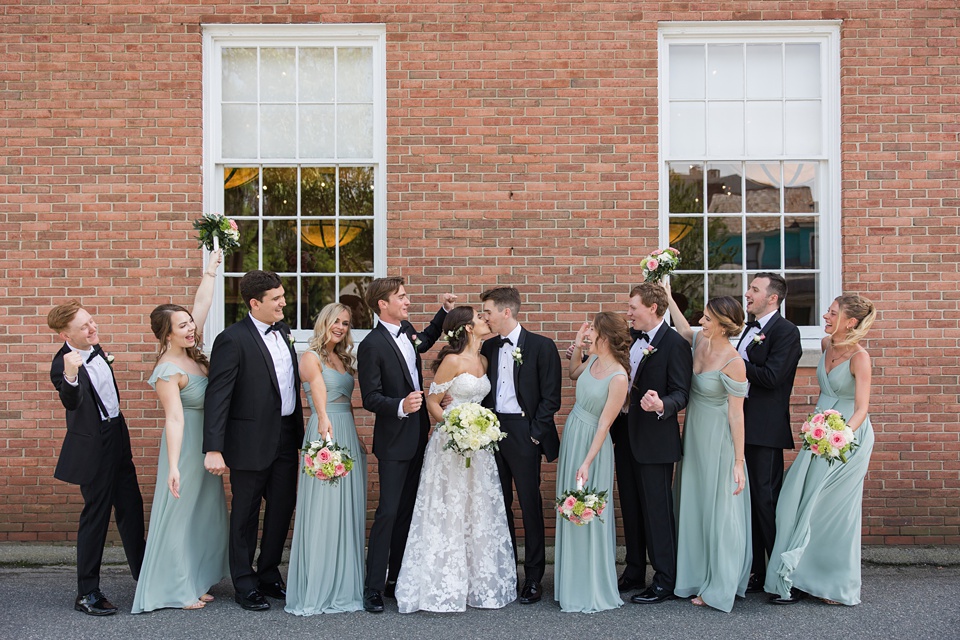This detailed photograph captures a joyful moment outside a reddish-brown brick building during a wedding celebration. The scene prominently features the bride and groom in the middle, sharing a kiss. They are surrounded by their bridal party, comprising six bridesmaids in seafoam, floor-length dresses and six groomsmen in black tuxedos. The bridesmaids enthusiastically hold up their flowers while everyone smiles and cheers. The bride is radiant in a strapless, white lace gown, adorned with flowers in her hair and holding a large white bouquet. The background reveals a red brick wall accented by two white-trimmed glass windows, with shades covering the top halves. The natural light suggests that the photo was taken in the late afternoon or early evening, possibly after the ceremony, capturing the vibrant and celebratory atmosphere of the occasion.